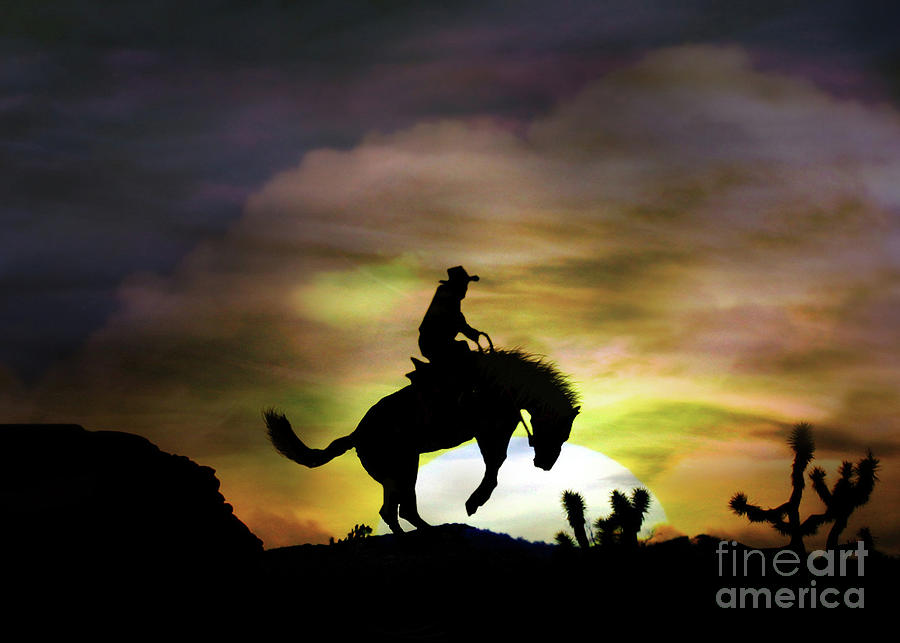In this captivating scene, either a photograph or a painting, the vast western landscape is serenely illuminated by a dramatic sunset. Across the bottom right corner, a subtle gray text reads "Fine Art America," confirming its artistic nature. The image is dominated by deep, dark silhouettes: a cowboy in a wide-brimmed hat clings to the reins of a horse caught in mid-buck, its front legs raised and head bent low. The background reveals the expansive Rocky Mountains, further accentuated by sparse, shadowed cacti.

The sky above showcases a stunning gradient—near the horizon, intense shades of dark orange and yellow melt into each other, painting the clouds in a mix of dusky blues and purples. A massive, pale white sun hovers just above the mountains, casting its last light over the scene. Higher up, clouds reflect a blend of yellow, pinkish, and beige hues, while the upper reaches of the sky transition into a rich dark blue. Overall, the image captures the raw, untamed beauty of the American West, frozen in a moment of dynamic tension and natural splendor.